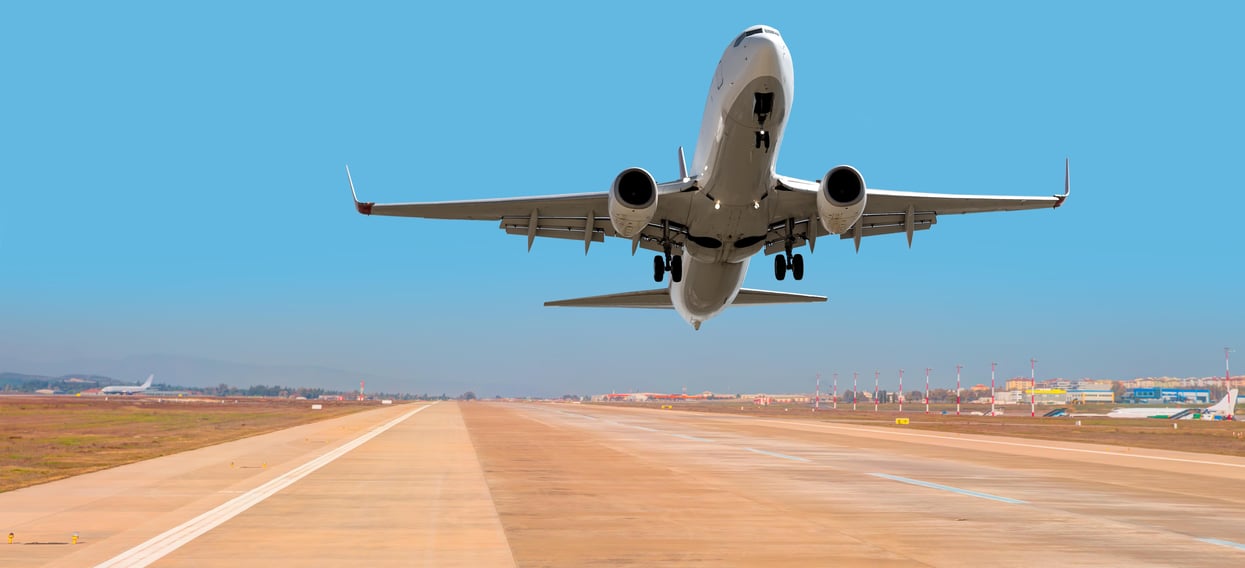The photo captures a large Delta airplane just taking off from a wide, long airfield with its landing gear still down. The airstrip, positioned in what appears to be a desert-like environment, is colored in light orange and beige with distinct white lines marking the sides and an interrupted line down the center. In the far distance, additional airplanes and various buildings are visible along the horizon, which is framed by mountains and trees. Above, the sky is a vast expanse of clear blue, punctuating the scene of early ascent. The bottom of the gray and white aircraft is prominently shown as it begins to lift, indicating the start of its flight from this bustling airfield.